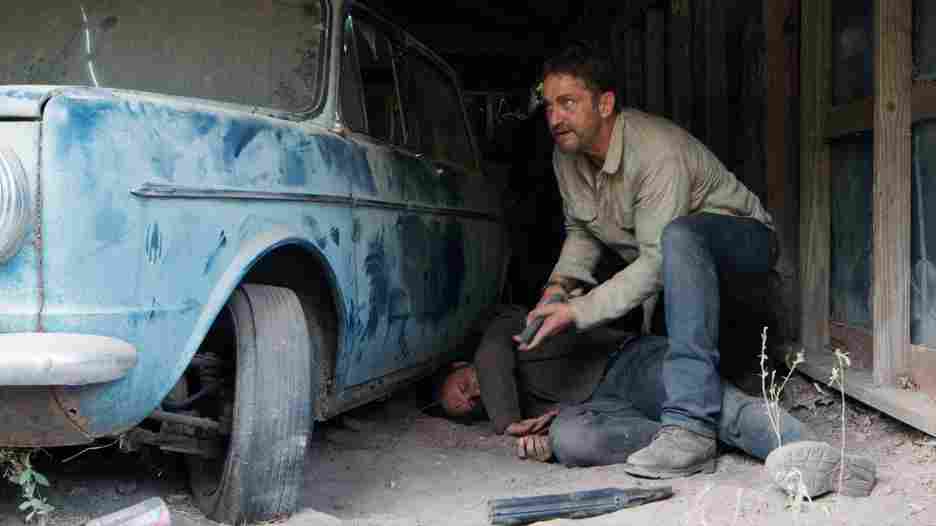The image depicts two men beside an ancient, dilapidated car, possibly from the 1960s or 70s, that is light blue with patches of darker blue, covered in dust and grime, some of its paint worn off, and its windshield clouded with dirt. The scene is set within a crumbling, rustic shed, discernible by the wooden beams and a window devoid of curtains in the background. The car appears non-functional, with rust spots and an undergrowth of weeds around its base. On the right side of the image, one man lies in the dirt, eyes closed, potentially injured or dead. He is clad in a gray long-sleeve shirt, blue jeans, and boots. His body is partially curled, with one leg bent underneath the other. Hovering over him is another man, dressed in blue jeans and a beige long-sleeve collared shirt. This man has short brown hair and a tense demeanor, looking off to the side, as if wary or hiding from someone. He is crouched with one knee on the ground and holds a gray object in his hand, possibly a gun. In front of him lies a small, unidentified black object, adding to the air of mystery and tension in the scene.